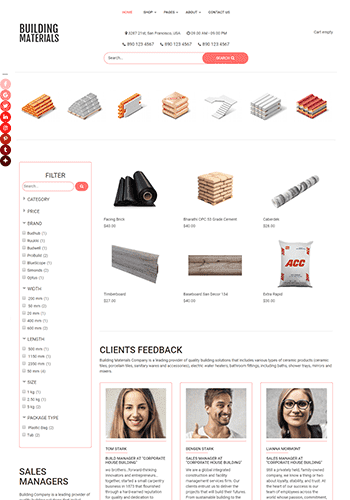**Detailed Caption:** 

The image showcases a screenshot of a simple e-commerce website dedicated to building materials. The background of the site is predominantly white, providing a clean and straightforward design. At the very top, the website is marked with the title "Building Materials" prominently displayed.

On the left side of the top navigation bar, there are several buttons. Most of the text on this navigation bar is black; however, some elements, like the 'Home' button, are highlighted in red. Despite slight blurriness, the navigation menu appears to include options like "Home," "Shop," "About Us," "Contact Us," and possibly other items that are not entirely legible.

Centered beneath the navigation bar is additional information, which may include a phone number and a search box designed in red. The search box features a red button labeled either 'Search' or similar. On the right side of this section, there is a cart icon with the label "Empty," likely linking to the shopping cart page.

Moving further down, the main content includes a display of some of their products. These products aggregate in the center of the page and appear to be either bricks or wood, though the exact material is vague due to the photo's quality. There are about five or six product images aligned horizontally, situated three to four lines from the top center of the screen.

On the left side is a filtering box for products, allowing users to sort items by criteria like length, size, category, and other attributes.

Below the featured products section, there are three more product images, bringing the total to about six. Towards the bottom of the page, there's a section titled "Client’s Feedback," followed by three informational boxes, although the content is not fully visible in the screenshot.